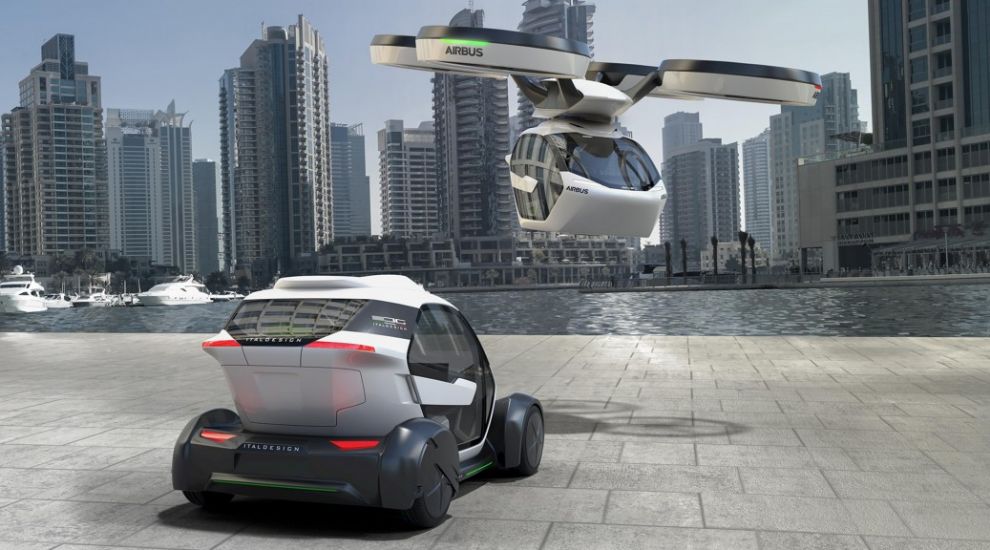In this AI-generated, photorealistic image, we see a futuristic urban setting dominated by a sleek cityscape with numerous skyscrapers. In the foreground, a cutting-edge, egg-shaped car with full glass doors and four wheels sits parked on a flagstone plaza. Above this car hovers an advanced passenger drone branded with "Airbus," featuring smoky plexiglass sides, white and flat black highlights, and distinctive green and red glowing strips on its front turbofans. The drone appears designed for human transportation, hinting at a future of aerial public transit. The backdrop includes a water harbor with several boats and yachts, adding a maritime charm to the ultra-modern city vibe. This scene, possibly from a show like Westworld, showcases a seamless blend of advanced vehicle technology and an expansive, futuristic metropolis.